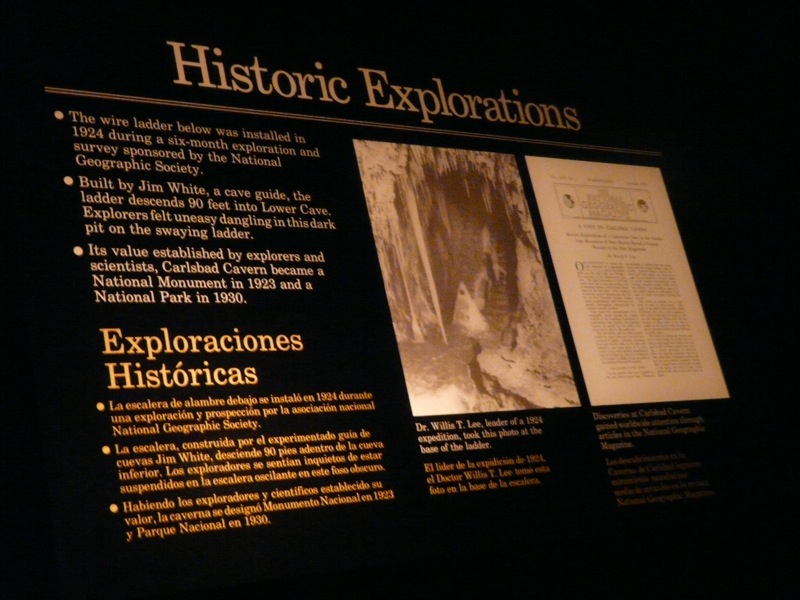This is a photograph of a museum display with a black background and gold lettering. At the top center, the display reads "Historic Explorations." Below this heading, on the left side, there is detailed text: "The wire ladder below was installed in 1924 during a six-month exploration and survey sponsored by the National Geographic Society. Built by Jim White, a cave guide, the ladder descends 90 feet into Lower Cave. Explorers felt uneasy dangling in this dark pit on the swaying ladder. Its value established by explorers and scientists, Carlsbad Cavern became a National Monument in 1923 and a National Park in 1930." This information is followed by a Spanish translation labeled "Exploraciones Históricas." 

To the right of the text, there is an old black-and-white photograph depicting the entrance to Carlsbad Caverns, with a person ascending a wire ladder. Next to the photograph is a white area containing an article and other historical documents, though they are out of focus and illegible in the image.